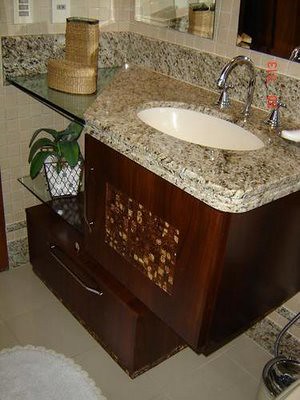The photo showcases a stylish bathroom with a focus on the sink area. The elegant marble countertop extends across the space, with a small basket or holder placed on the left, providing a touch of organization. The right side of the counter features a pristine white sink equipped with a sleek silver faucet that gracefully curves over it. The faucet is complemented by two matching silver handles. Below the countertop, there's a glass shelf holding a small, green plant, adding a refreshing element to the scene. Directly beneath the sink, a cabinet with a handle provides concealed storage, while a drawer with a large central handle occupies the bottom section. The floor is adorned with clean white tiles and a matching white mat, completing the polished look of the bathroom.